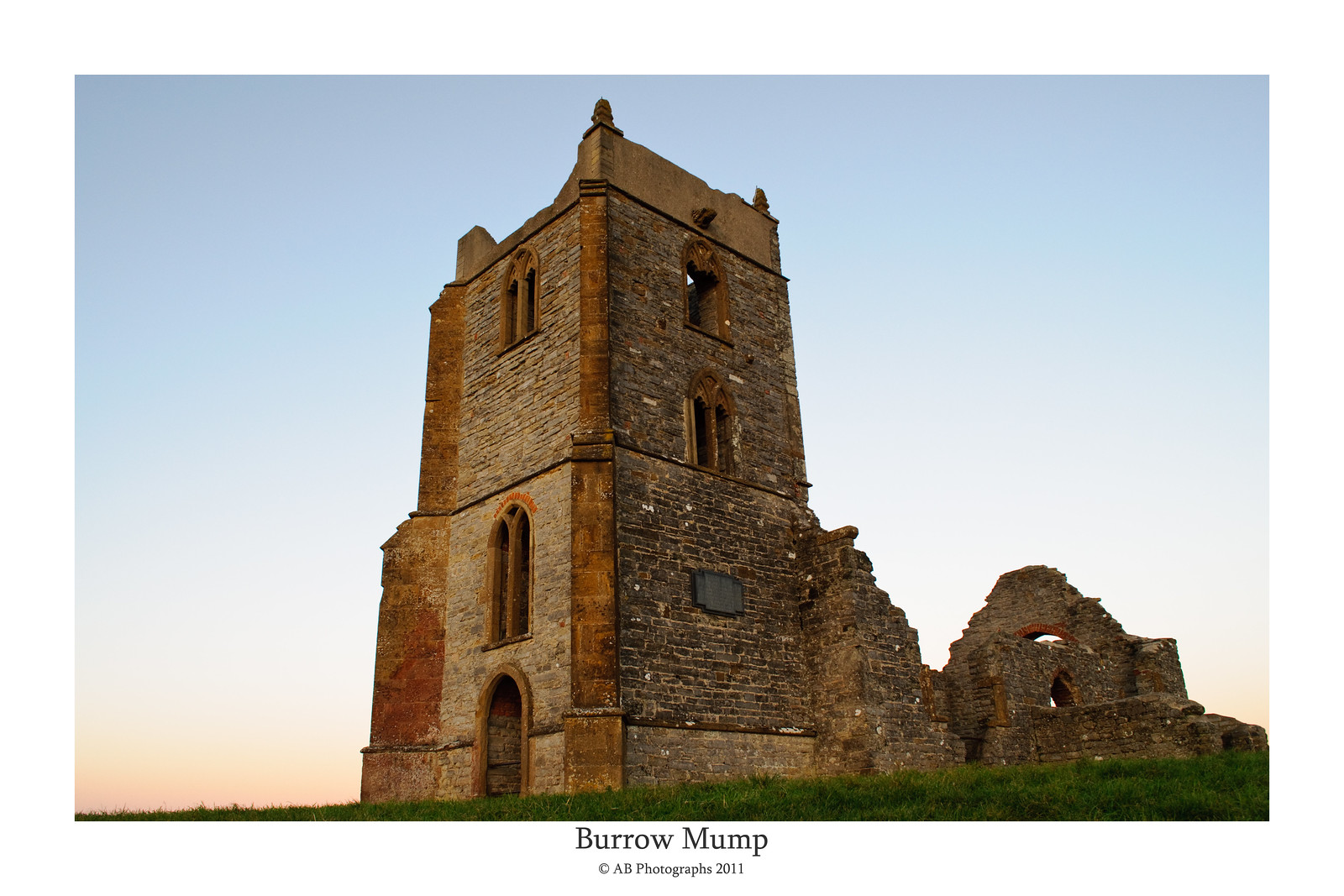This photograph captures the crumbling remnants of what appears to be an ancient ruin, situated on a grassy field under a clear blue sky. Dominating the left side of the image is a primarily intact tall section, which looks like it was once a tower. The structure, composed of brick and stone in varying shades of dark brown, light brown, and tan, features a series of arched windows and an arched doorway at the bottom of its left wall. To the right, the building descends into disrepair, with its walls reduced to broken bases and scattered fragments, revealing additional archways amidst the ruins. The sky above transitions from deep blue to a lighter hue with hints of pink and white near the horizon, suggesting the scene might be set at sunset or sunrise. A white border at the bottom of the photograph bears black text: "Burrow Mump, AB Photographs, 2011."